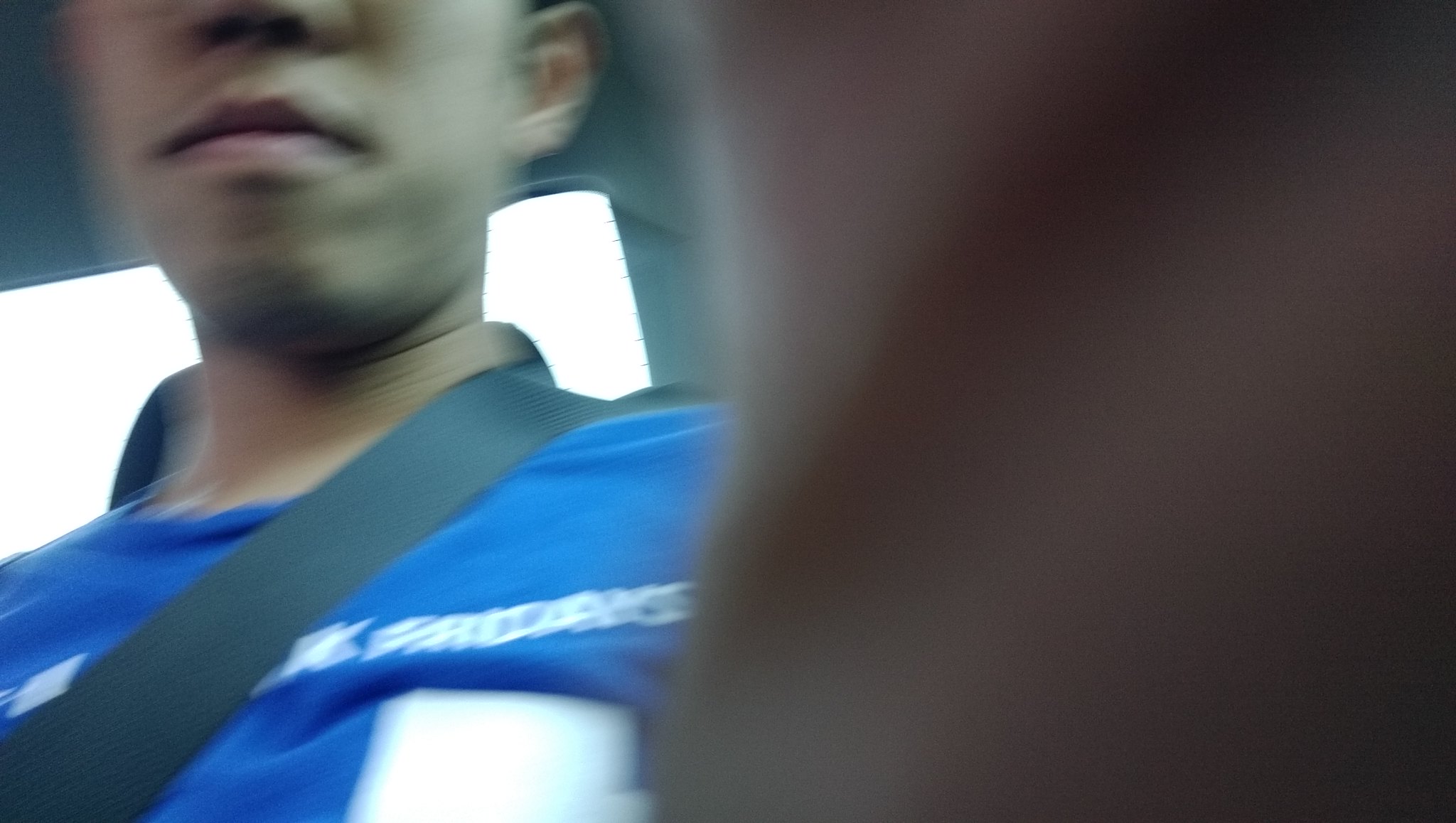This detailed photograph captures an accidental selfie of a male figure in a vehicle during daylight. The image, in landscape mode, shows the person seated, though it's unclear whether he occupies the driver's or passenger's seat. The photo is a close-up, revealing only the lower part of his face from the nostrils downward, including the top of his left ear, and notably includes his round face and lips, suggesting he is of Caribbean or possibly South American descent with brown skin. 

He is wearing a blurry blue t-shirt with some indistinct white lettering, possibly a number, which suggests it might be a football top. A black seat belt runs diagonally over his left shoulder, extending down to the left corner of the image. Behind his blurred head and torso, a headrest and a window are somewhat visible, affirming he is indeed in a car. The entire right side of the image is obscured by a flesh-colored blur, likely his palm covering the lens, indicating he is holding the camera or phone and accidentally took the selfie.